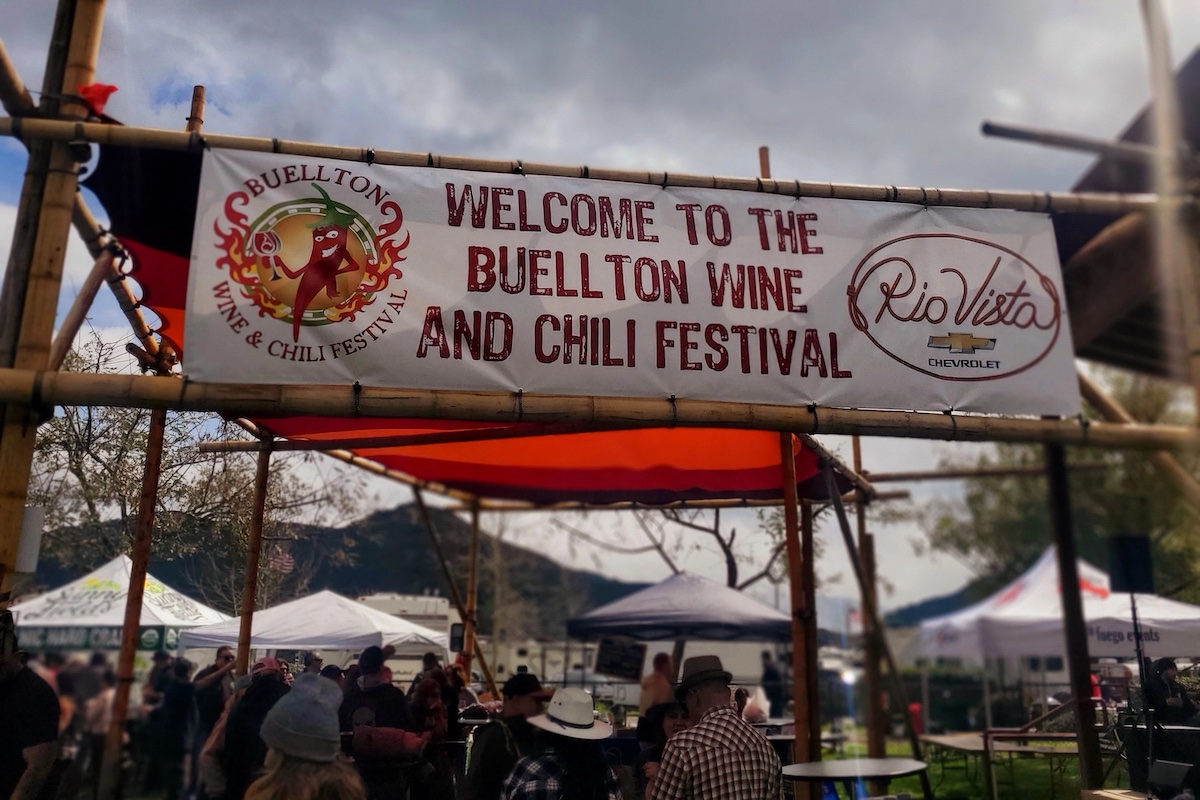This photograph captures the bustling atmosphere of the Buellton Wine and Chili Festival. Dominating the scene is a long white banner attached to horizontal poles supported by vertical ones. The banner reads, "Welcome to the Buellton Wine and Chili Festival" in the center, and prominently features a cartoonish red chili pepper with a green top hat, eyes, and a mouth, holding a glass of wine. The chili pepper is surrounded by red flames and appears within an orange circle bordered by green lines. To the left, "Buellton" is written in curved letters above the pepper. To the right, in cursive letters connected as if by a red lasso, is "Rio Vista," followed by the Chevrolet logo and branding.

The festival scene below is vibrant, with numerous pop-up tents and awnings of varying sizes. Beneath these structures, attendees, some wearing cowboy hats and fedoras, gather around high-top tables. The grounds are lush with green grass and leafy trees, indicating a spring or summer setting. The sky above is cloudy, adding a soft light to the lively crowd. In the background, rolling hills frame the event, enhancing the picturesque quality of the festival. The festival appears well-attended, with people standing by the tents, presumably sampling various types of chili and possibly other treats, making it a lively and communal gathering.